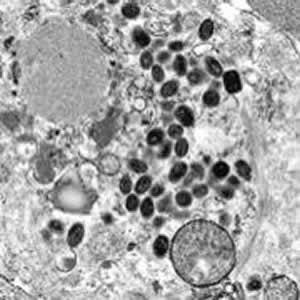This black and white microscopic image captures a detailed cellular structure at an intricate level. At the center of the image, numerous spherical dark circles can be observed, each surrounded by lighter shades of gray and white, creating a striking contrast. These spherical objects, appearing to float within a semi-opaque medium, suggest a densely packed environment. Additionally, among the primary spherical formations, there are several more varied shapes—some round, others more oblong—all maintaining roughly similar dimensions. The precise scale remains ambiguous due to the nature of the microscopic capture, but this image likely depicts cells or cellular components suspended within a biological or scientific medium, highlighting the complexities and detailed textures observable only through high-magnification microscopy.